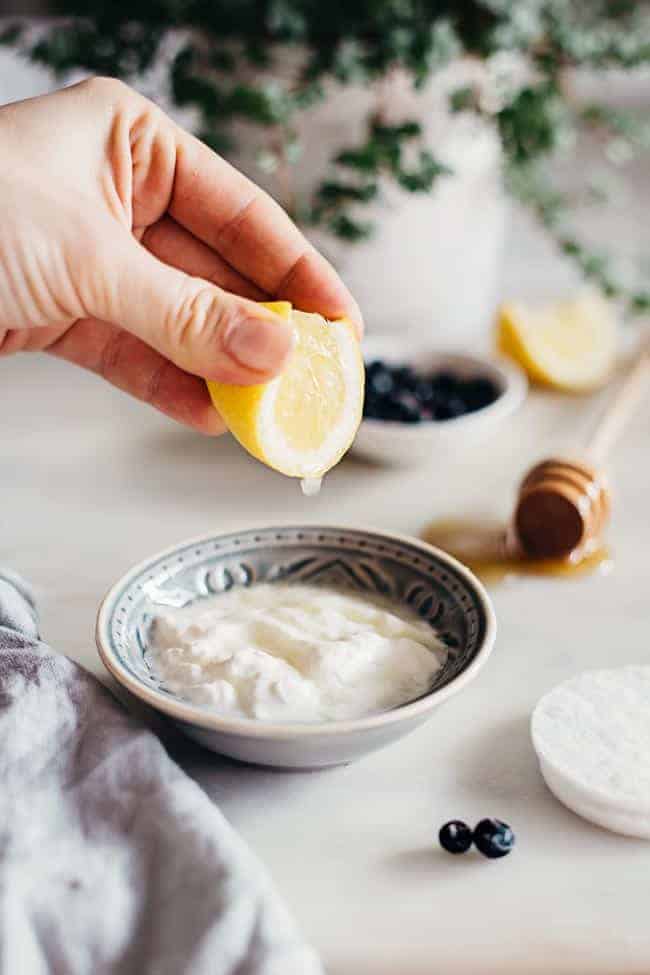The indoor, vertically rectangular, full-color photograph appears meticulously staged, capturing a culinary scene. In the upper left corner, a Caucasian left hand is squeezing a lemon wedge over a small white and blue ceramic bowl, likely containing yogurt or sour cream. Central to the image is a white bowl filled with blueberries, accompanied by another lemon wedge. In the lower right corner, a couple of blueberries are visible near two stacked white objects, possibly pads or coasters. The upper right corner features a honey dipper with honey smeared around, placed on the table. At the top center, a white planter with a vibrant green fern adds a touch of nature to the backdrop. The primary focus is on the hand squeezing the lemon, with the rest of the elements slightly out of focus, creating a harmonious and detailed culinary setup.